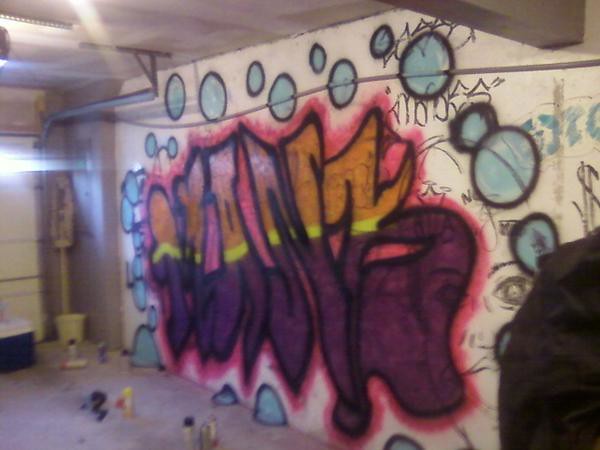In this photograph taken in an unfinished basement, the white-painted walls provide a stark backdrop to the scene, while the cement floor underscores the space's raw, industrial feel. The ceiling, also white, remains unadorned, lending a sense of openness to the otherwise enclosed room. In the top right corner, a partial view of a support beam hints at the structural elements holding up the space. The bottom right corner of the image captures the black sleeve of the photographer’s jacket, adding a touch of human presence to an otherwise static setting.

Dominating the wall is a piece of graffiti art that stands as the focal point of the image. The word "Manza" is vividly scrawled in a dynamic blend of colors: it starts with orange at the top, transitions to purple at the bottom, and is bisected horizontally by a bold, yellow stripe. Scattered around this central design are numerous blue bubbles, each neatly outlined in black, adding a playful and almost whimsical touch to the gritty environment. This juxtaposition of vibrant graffiti against the unfinished, utilitarian backdrop makes for an intriguing and visually stimulating composition.